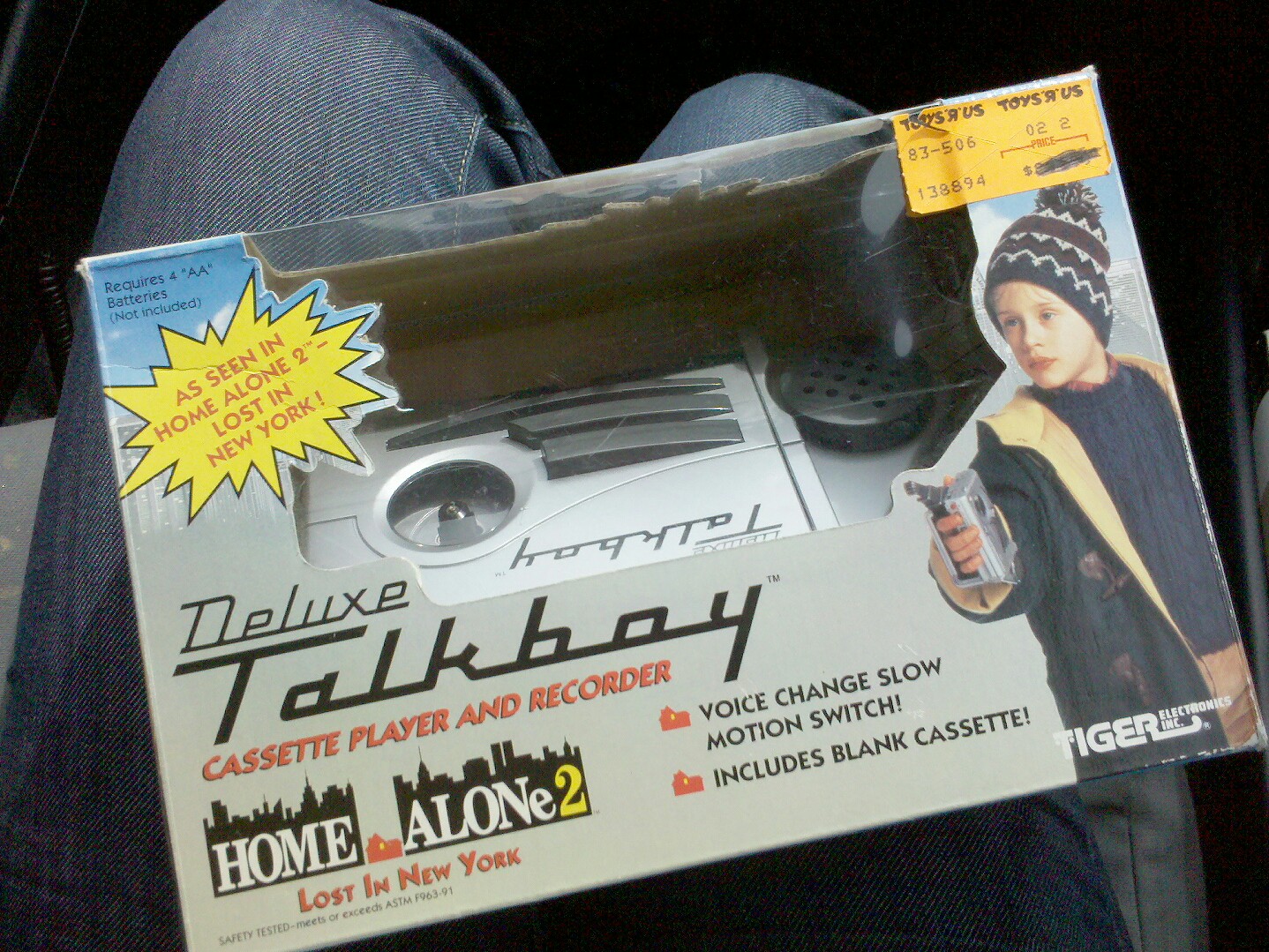The image depicts a slightly worn box of a Deluxe Talkboy Cassette Player and Recorder from Tiger Electronics, prominently featured in "Home Alone 2: Lost in New York." The box is sitting diagonally on a man's lap, who is wearing blue jeans, possibly seated in a car, given the visible gray seat. The packaging, predominantly gray with yellow highlights, also includes splashes of black, light blue, and orange. A picture of Macaulay Culkin from the movie is displayed on the right side, where he's holding the Talkboy, dressed in a blue jacket with a black and white ski cap, and black pants. The upper right corner bears a Toys R Us price tag, with the price crossed out. The box also features red lettering with a yellow starburst stating "as seen in Home Alone 2: Lost in New York," and details such as "Voice Change Slow Motion Switch" and a note that it requires four AA batteries, which are not included. The setting suggests a dark-lit room with the box clearly at the center of the image.